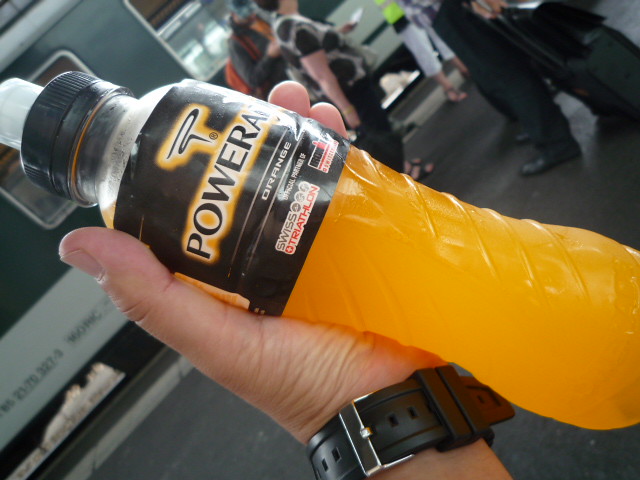In a landscape-oriented photograph, a man's hand prominently holds up an orange Powerade sport bottle. The sleek, ergonomically designed bottle features the distinctive black Powerade logo set against an orange and white background. The flavor is orange, indicated by white text on the label. The bottle also boasts sponsorships, with logos indicating official partnerships with Swiss Triathlon and Ironman. The Powerade bottle appears completely full and unopened, capped with a black sport cap that includes a nozzle sealed by a clear plastic covering. 

The man holding the bottle wears a sturdy watch with a silver-toned buckle, the watch band measuring nearly an inch wide. 

In the background, various figures contribute to the setting, lending context to the scene. The immediacy of first responders is suggested by visible pants and shoes. A woman in black pants, sandals, and a cow print top can be seen. Additionally, there's a small child dressed in a high-visibility yellow vest and white pants with sandals, only partially visible. Another man stands out, wearing an orange backpack, looking down with a bandana tied around his head. In the distance, a train car rests on tracks, implying that the scene takes place at a train station.